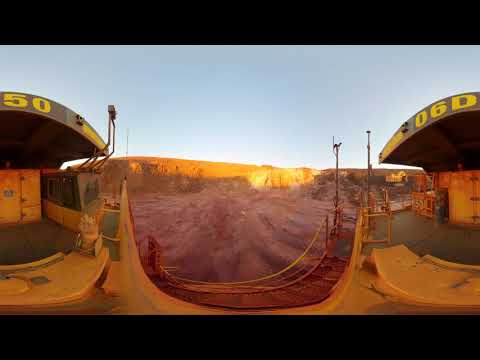The image appears to be a distorted view of a building, possibly a gas station or a refinery, situated in a deserted, desert-like area. Notably, the roof of the structure displays large, yellow numbers reading "5-0" on the left and "0-6-D" on the right. What stands out in the scene are peculiar poles with attached gadgets, suggesting equipment for surveying or recording purposes, possibly cameras.

The image showcases a strange visual phenomenon where the building seems duplicated on the left and right sides, likely due to a photographic distortion. In the backdrop, a vast expanse of deserted land is visible, featuring patches of grass and a dirt path that might be steps or a skateboard ramp leading into the distance. The ground reflects an orangey-brown hue, adding to the desolate ambiance.

The sky above is clear and blue, indicating a sunny day. Shadows and light patterns suggest the image was taken during daytime, with some indications of a setting sun casting long shadows across the scene. Enhancing the surreal quality, the perspective might be from a bridge-like structure overlooking a canyon or crevasse, adding to the image’s disorienting feel.